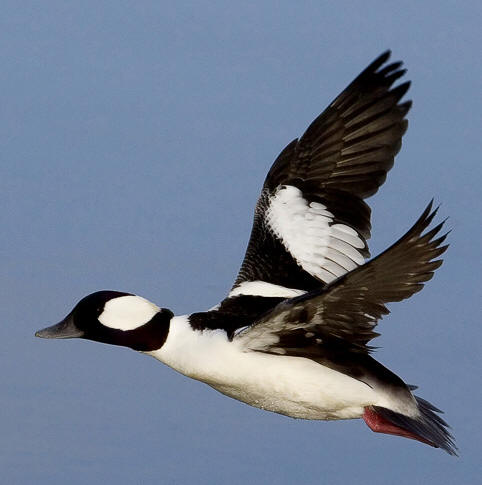This close-up photograph captures a Bufflehead duck in mid-flight, set against a smooth, grayish-blue sky. The duck is seen from the side with its wings extended upwards in a V-shape. The bird features distinct coloration: a black head transitioning to a white patch behind the neck, followed by a black collar-like band around the neck. Its underbelly is white, while its back remains predominantly black. The wings are striking, with a central white patch contrasted against the black feathers, which merge into a very deep rust color towards the front edge. The bird's webbed feet are tucked in, showing a pinkish-red hue. The photograph is predominantly vertical, highlighting the bird as the sole subject without any accompanying text or additional elements in the frame.